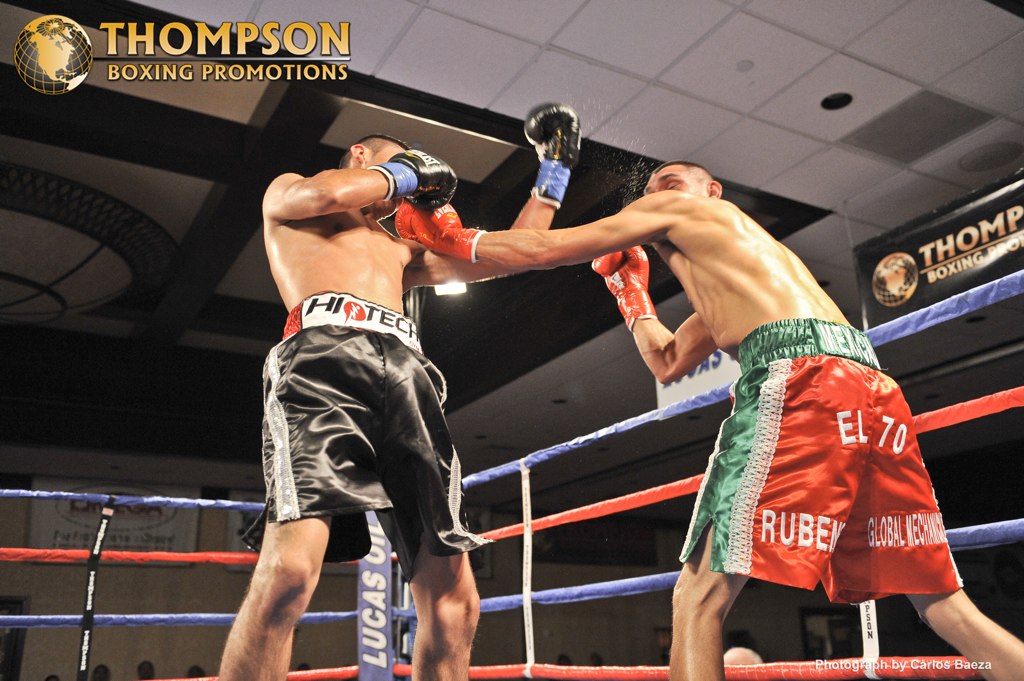This vibrant color photograph captures an intense moment inside a boxing ring, showcasing two men engaged in a fierce match. The image is endorsed by Thompson Boxing Promotions, which is prominently displayed in the top left corner, indicating it as an official promotional photograph. A banner for Thompson Boxing adorns the right-hand side of the photo, featuring their logo—a black and gold globe. The boxing ring itself is colorfully outlined with alternating blue and red ropes.

In the foreground, the contender on the left is dressed in long black boxing trunks with the name "Hi-Tech" emblazoned around the waistband, complemented by matching black boxing gloves. His opponent, positioned on the right, sports vibrant red, green, and white shorts with "Mexico" proudly displayed on the waistband. His attire is detailed further with "EL-70," "Rubin," and "Global Mechanics" inscriptions. He also dons coordinating red boxing gloves. Both fighters are shirtless, embodying the raw intensity of the sport.

This action-packed photo captures the climactic moment as both athletes throw powerful punches, embodying the spirit and adrenaline of a high-stakes boxing match.